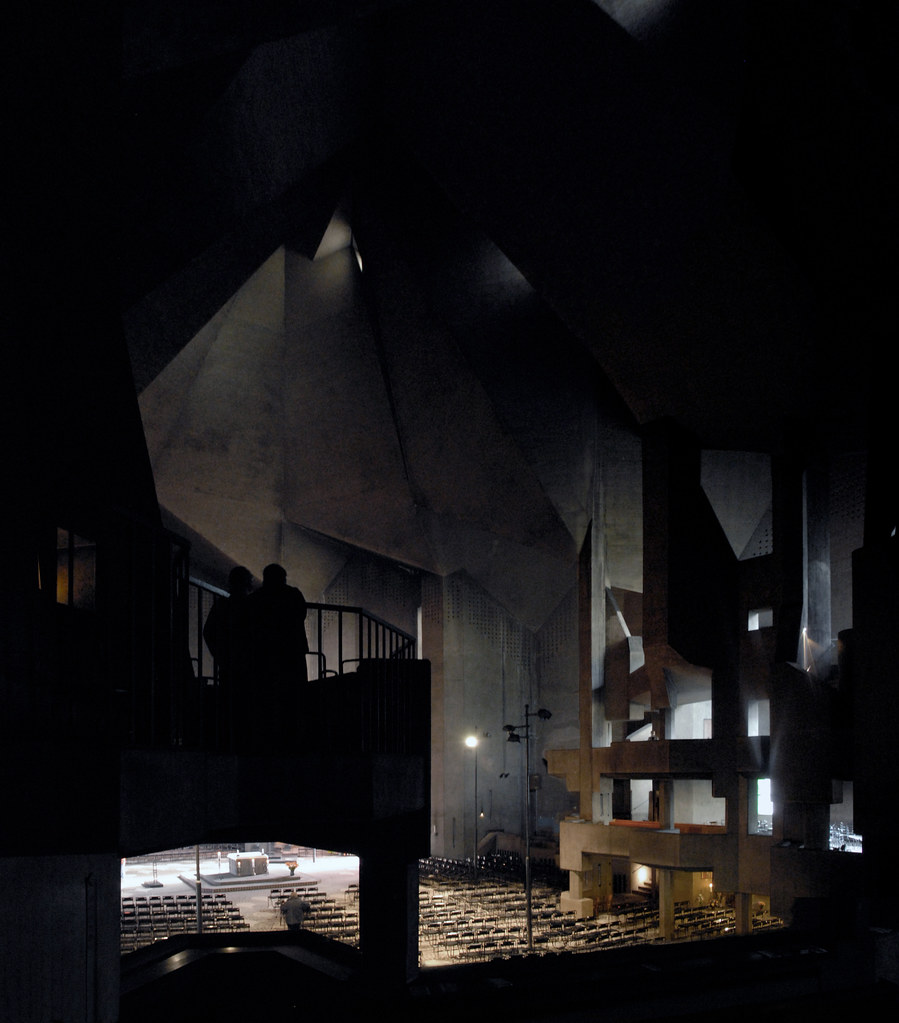In this dark yet evocative black-and-white photograph, the interplay of light and shadow creates a dramatic scene. The foreground features the silhouetted forms of two individuals standing on a balcony located at the bottom left corner of the image. The balcony, with its prominent railing, is part of a concrete building that appears elevated above the ground. To the right, the concrete walls of the building rise vertically, showcasing three distinct, blocky stories, each with its own balcony. Dim light seeps from behind these balconies, adding depth to the scene.

Directly below these balconies, in the center foreground, numerous foldable metal chairs are scattered, perhaps suggesting a gathering of everyday people. To the bottom left, a well-lit pedestal stands out, surrounded by two steps outlining a rectangular area, casting a stark contrast to the otherwise dark surroundings. The building itself ascends into a cone at the top center of the image, evoking the atmosphere of a cult or religious sanctuary. The composition, with its varied elements and intense contrasts, captivates and intrigues, inviting viewers to delve deeper into the story being told.